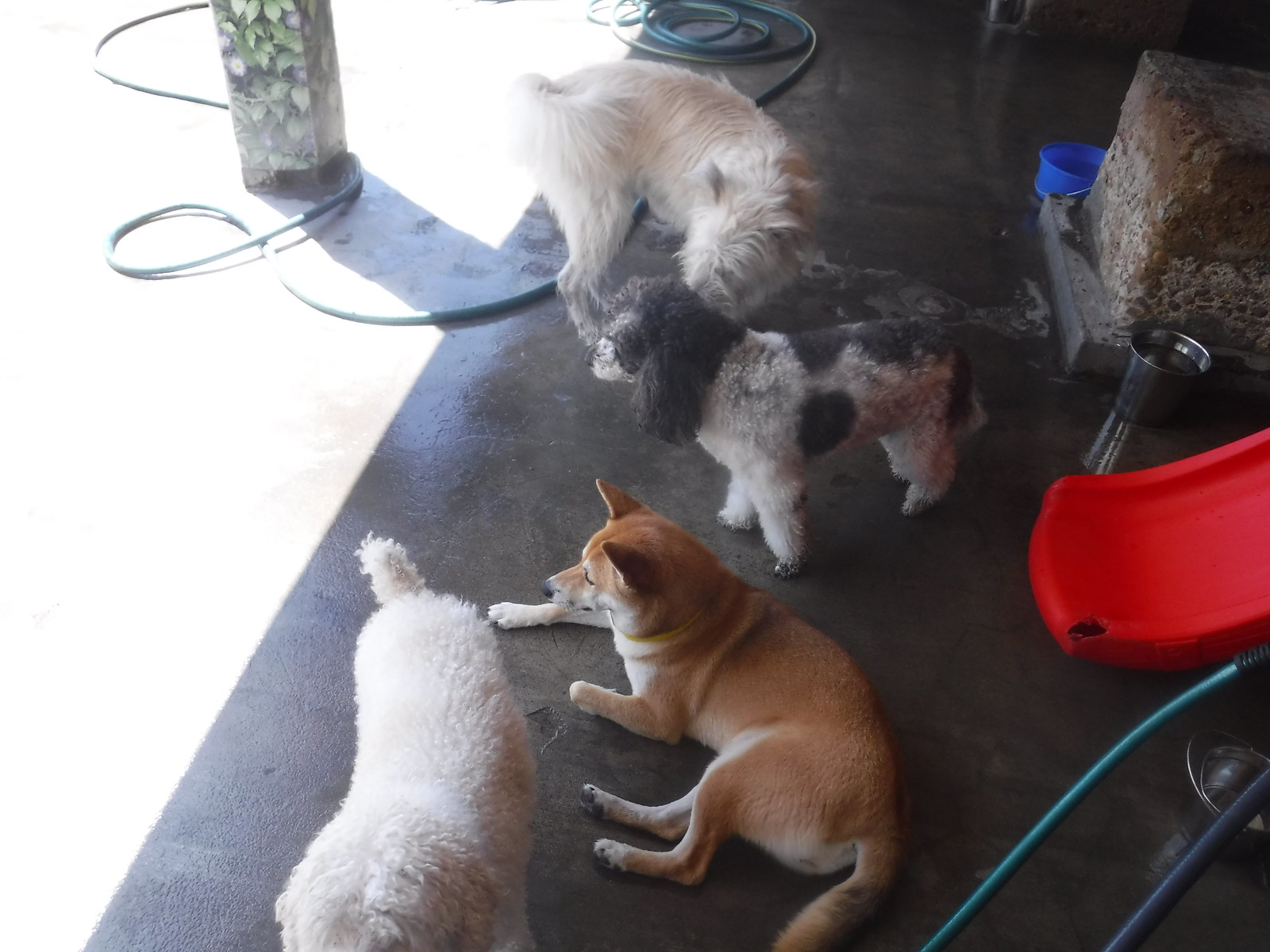This color photograph captures a group of four dogs on a sunlit concrete slab under the partial shade of a covered patio or structure. A stark dividing line of bright, almost blinding, sunlight cuts diagonally from the bottom left to the midway point at the top of the image, casting a sharp contrast with the shaded area on the right. A support pillar, wrapped in green leaf-patterned paper, stands prominently in the bright wedge of sunlight, with a garden hose looping around it and extending into the shadowed area.

To the right of the frame, partially visible in the shade, is the bottom portion of a red plastic toddler slide. Nearby, a blue water dish rests on the ground. Also visible is a big concrete block, possibly the base of another pillar.

The four dogs are gathered in the shaded part of the image. Starting from the left: a white, fluffy dog with its head slightly cropped out of the frame; next, a tan Shiba Inu lying down with its pointed ears alert. Standing behind the Shiba Inu is a white dog with black spots, presumably a poodle mix. The last dog resembles a Westie but with longer legs and a fringed tail, looking like a terrier of some sort. These dogs seem relaxed yet attentive, with the brown Shiba Inu particularly focused, gazing intently towards the sunny area.